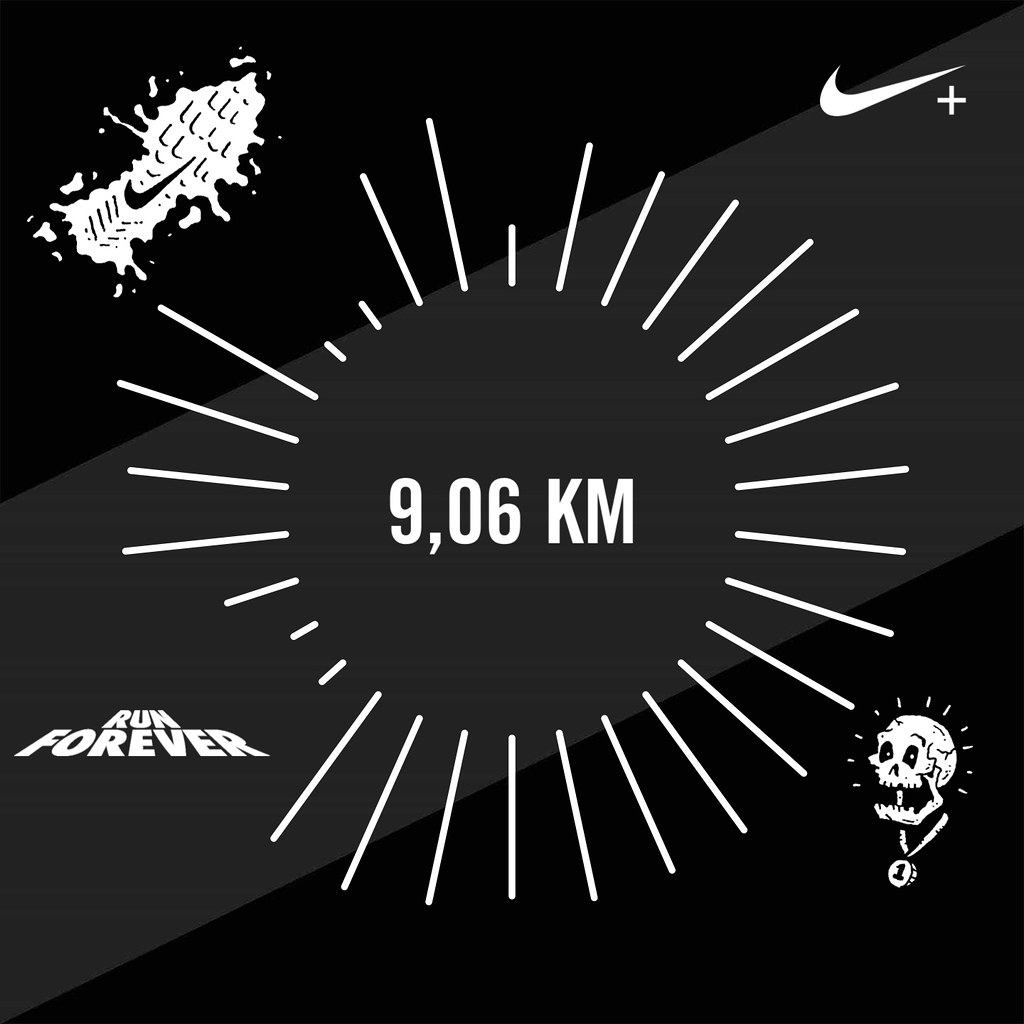This striking digital illustration features a central focal point where the text "9,06 KM" is prominently displayed, surrounded by lines of varying lengths radiating outward, giving the impression of sun rays without a defined central circle. The overall background of the image is black, bisected by a gray stripe from the bottom left corner to the top right corner.

In the top left corner, a splatter effect resembling a shoe print contains a black Nike logo. The top right corner showcases another Nike logo in white, accompanied by a plus sign. The bottom left corner features the text "Run Forever" in a font reminiscent of the Star Wars credit sequence, while the bottom right corner displays a skull wearing a medal with the number 1, with lines emanating from its face that mimic the design in the center of the illustration. The combination of these elements creates a visually dynamic and cohesive design centered around the theme of running and achievement.